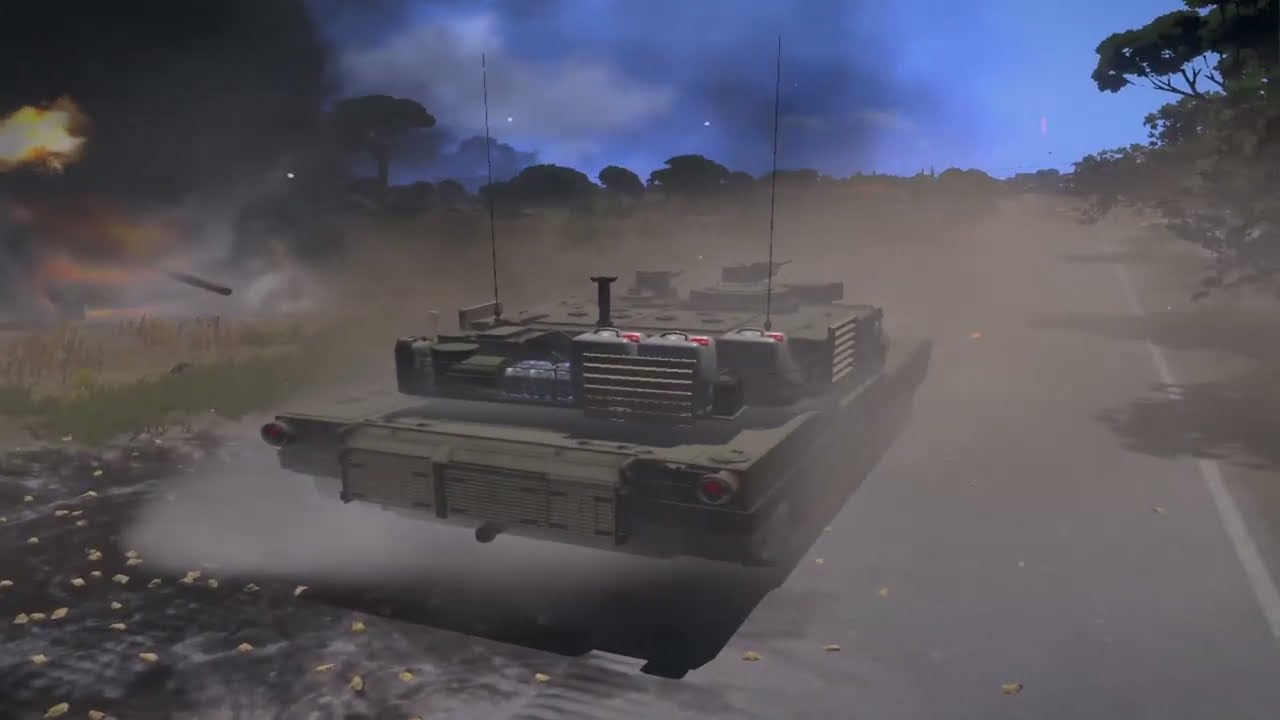The image is a chaotic scene likely captured from a war-themed video game. Dominating the center is a huge, greenish military vehicle that resembles a tank, adorned with multiple turrets, compressors, and two prominent antennas on either side. This formidable machine is speeding down a gray road marked by a white line on the right and is actively engaged in combat, evidenced by a large gun barrel and a smaller gun turret at the front. On the left, a black artillery piece targets the vehicle, producing a black streak that cuts across the smoky, cluttered air.

The environment is darkened by extensive black smoke, particularly concentrated in the upper left corner, where an explosion or fire adds a reddish hue to the chaotic foreground, littered with debris. Despite the gloom, patches of blue sky and white clouds are faintly visible behind the smoky shroud. The road is flanked by trees on both sides, which appear partially obscured and distorted by the pervasive smoke. The scene conveys a vivid impression of a war zone, intensified by the combination of visual elements such as the speeding tank, the artillery fire, and the billowing smoke, immersing viewers in its gritty, high-stakes atmosphere.